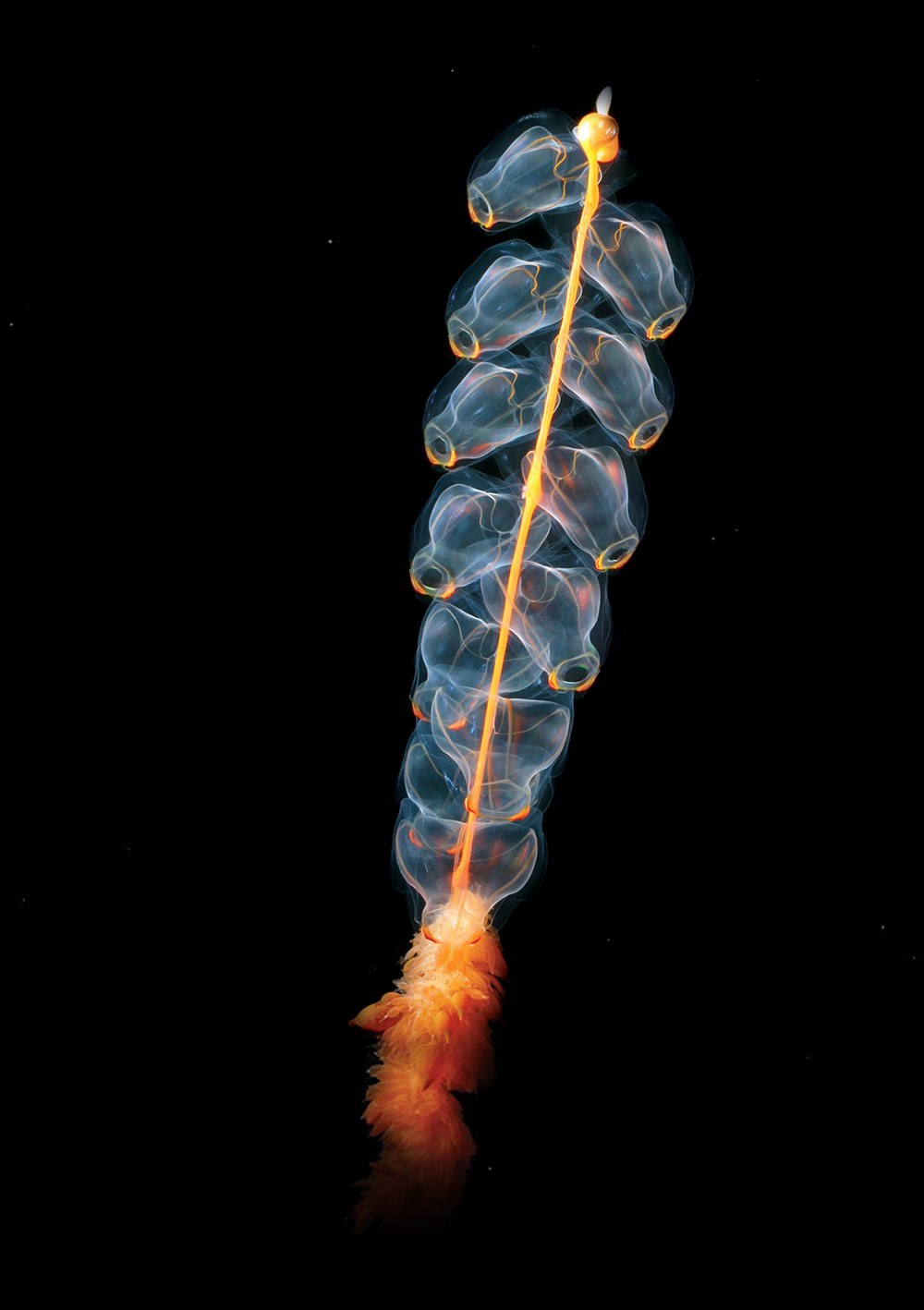The image depicts a striking invertebrate known as a Siphonosphora, set against a stark black background, potentially enhanced with black light to highlight its vivid, neon colors. Central to the composition is a long, yellowish column that culminates in a small orange bulb at the top. Flanking this central column are eight translucent, tulip-like structures, four on each side, resembling closed flower buds or amphorae turned on edge. These structures have circular, clear ends that are tinged with orange, giving them a liquid-like appearance. Descending from these, there are three larger, almost bubble-like formations before reaching an orange and red mass at the bottom, which seems feathery in texture. The overall impression is that of a luminescent sea creature, possibly photographed underwater, emitting bright and vivid hues that make it appear almost otherworldly.